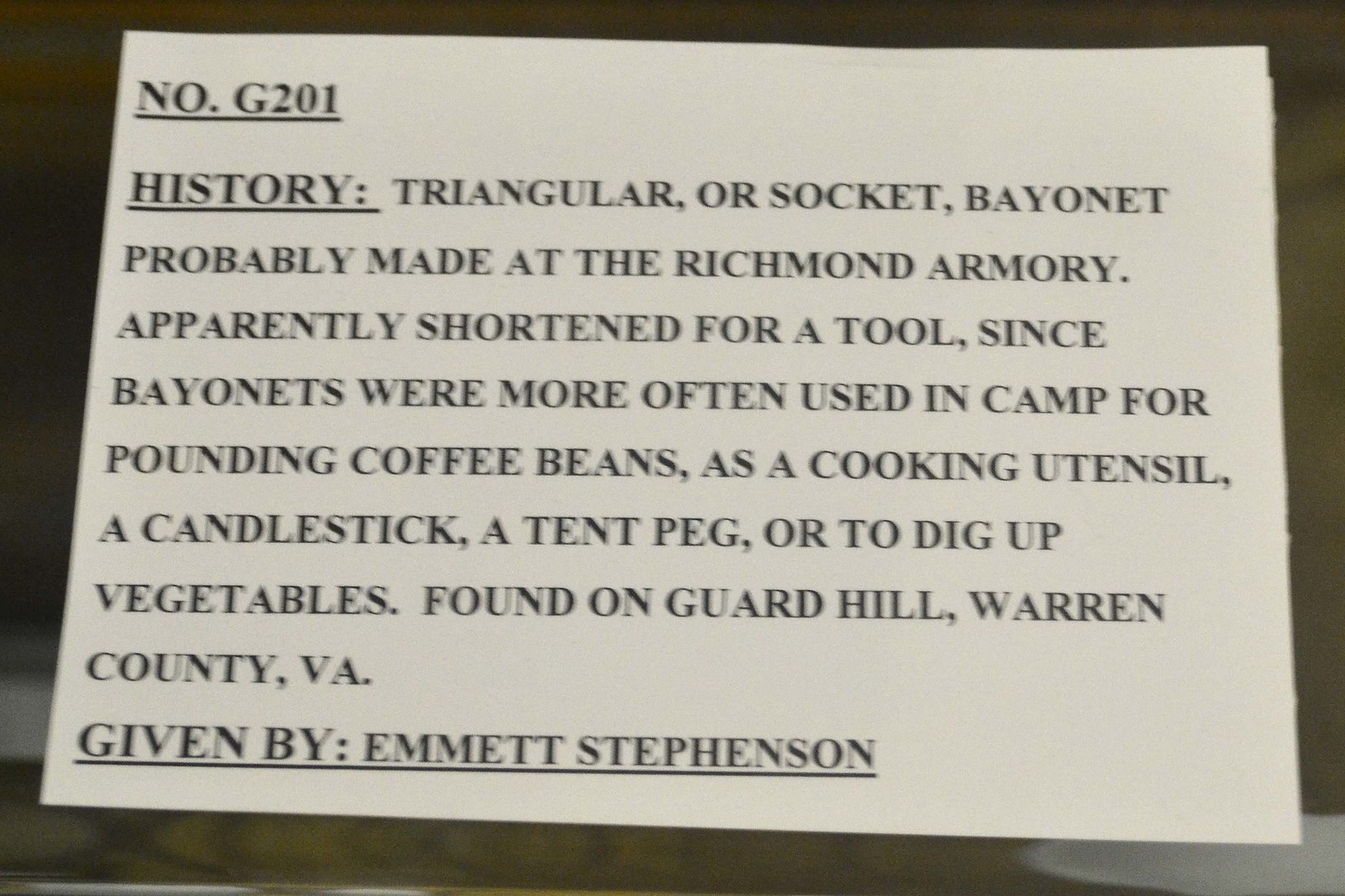The image is a horizontally aligned, somewhat blurry photograph featuring a white rectangular piece of paper centrally positioned. The background is predominantly black along the top and sides, with a green and yellow mix towards the bottom, possibly resembling a counter top. The paper, slightly wider than tall, has a black underline under the top-left text, "NUMBER G201." Directly beneath, also underlined, is the word "HISTORY." The remaining lines are in all-cap black text, left-aligned, describing a "triangular or socket bayonet, probably made at the Richmond Armory." The bayonet appears to have been shortened for use as a tool, commonly utilized in camps for various purposes such as pounding coffee beans, functioning as a cooking utensil, candlestick, tent peg, or digging up vegetables. This artifact was "found on Guard Hill, Warren County, Virginia" and "given by Emmett Stevenson," with the donor's name underlined. The paper is surrounded by an approximately one-inch negative space border.